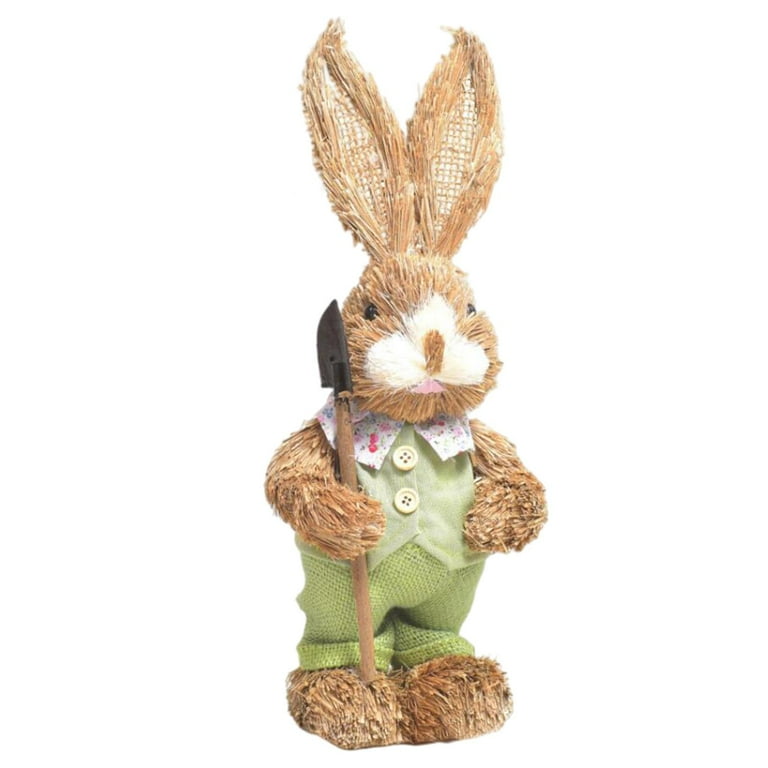The photograph captures an endearing stuffed bunny, likely an Easter decoration, standing upright against a white background. The bunny, constructed from a straw-like material, features a warm brown fur with a tufted white nose and mouth area, and a brown nose and pink mouth that add to its charm. Dark, marble-like eyes punctuate its expressive face. The bunny's tall and rigid ears, supported possibly by internal wires, reach towards the top of the image.

Dressed in an adorable green outfit, the bunny sports long woven or knitted pants and a buttoned-up vest, creating a cohesive and dressed-up look. The vest, a darker green, has two small green buttons and is layered over its pants to give an impression of an overall ensemble. A white collar adorned with a floral pink or red design encircles its neck, hinting at a playful, yet elegant style. In its right paw, the bunny holds a small gardening shovel, nearly as long as it is, contributing to the whimsical gardening theme. The overall presentation is one of delightful detail, perfect for evoking the springtime spirit.